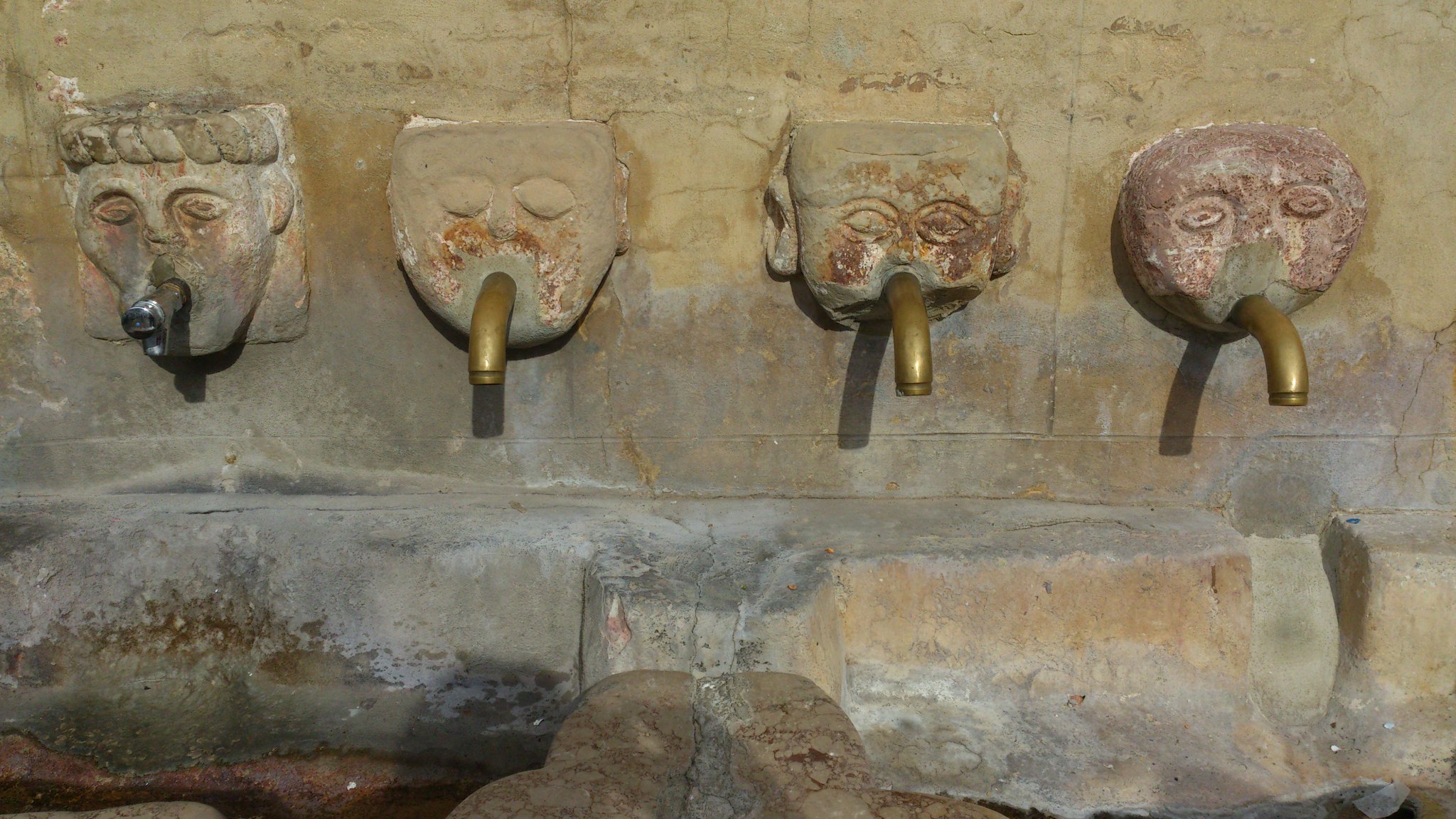This detailed color photograph, taken outdoors during the daytime, showcases a historic stone fountain set against an aged and weathered stone wall. The wall, displaying a rich palette of beige, gray, and greenish tones likely due to aging and mildew, features four intricately carved stone faces. These faces, embedded in the wall, function as faucets with water spouting from their mouths. 

Starting from the left, the first face has short, curly hair and a silver-colored metal spout extending from its mouth, accentuating its chiseled chin, prominent nose, and defined eyes and eyebrows. Moving to the second face, it appears less sharply defined with its eyes closed and a similar spout. The third face, distinguished by visible ears and open eyes, continues the pattern with another spout. Finally, the fourth face is carved from a slightly different, reddish rock, contrasting the predominantly brown faces and features a straighter spout.

The diverse expressions and shapes — round, square, and regular face-shaped — add character to the scene, providing a glimpse into the architectural style and functional artistry of the fountain, possibly used for draining water from the roof of what seems to be a very old building.